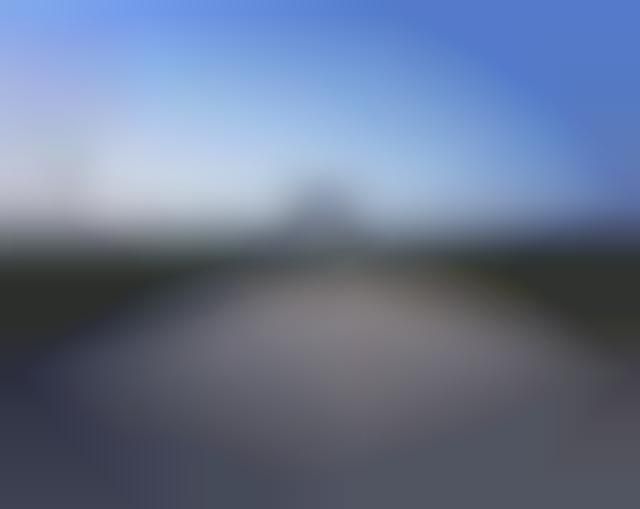In this blurry outdoor color photograph, the composition features an indistinct but discernible gradient of colors and shapes. At the bottom of the frame, there's a strip of dark to light gray, transitioning into a horizontal almond-shaped light gray to beige area. Flanking this almond shape, dark green triangular shapes extend slightly upward. Central to the image, approximately at the horizon line, a pale gray triangle emerges, neighbored by a strip of light blue to white. Overarching the top left of the frame is a blurred mix of very light pink to light gray, while the top right showcases a deeper blue gradient. Despite the heavy blur and lack of fine detail, the photo conveys a sense of a landscape with subtle color transitions and an indistinct horizon dividing lighter and darker tones.